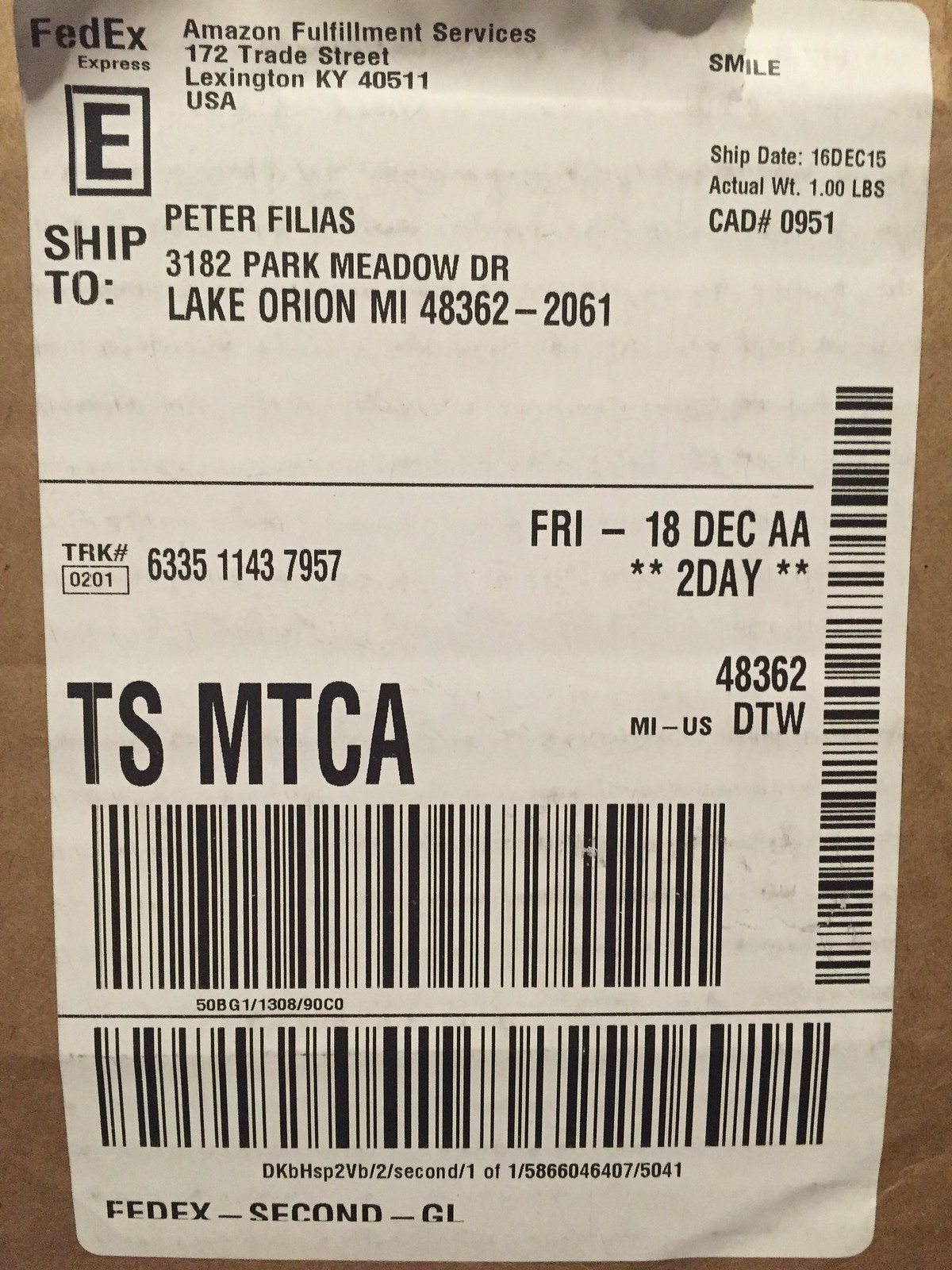This detailed image captures a shipping label affixed to what appears to be a cardboard box or brown paper envelope. The label prominently features the FedEx Express logo in the top left corner. It documents that the package originated from Amazon Fulfillment Services at 172 Trade Street, Lexington, KY 40511, USA, and is addressed to Peter Villiers at 3182 Park Meadow Drive, Lake Orion, MI 48362-2601. The shipment date is marked as December 16, 2015, and it was sent via two-day shipping, with the expected delivery date on Friday, December 18, 2015. The label displays several important details including three barcodes, a tracking number, and additional codes like "TS MTCA" in bold letters, along with a weight of one pound. The label is printed in black ink on a white sticker, typical for FedEx packages, containing various codes and numbers crucial for the shipment's logistics.